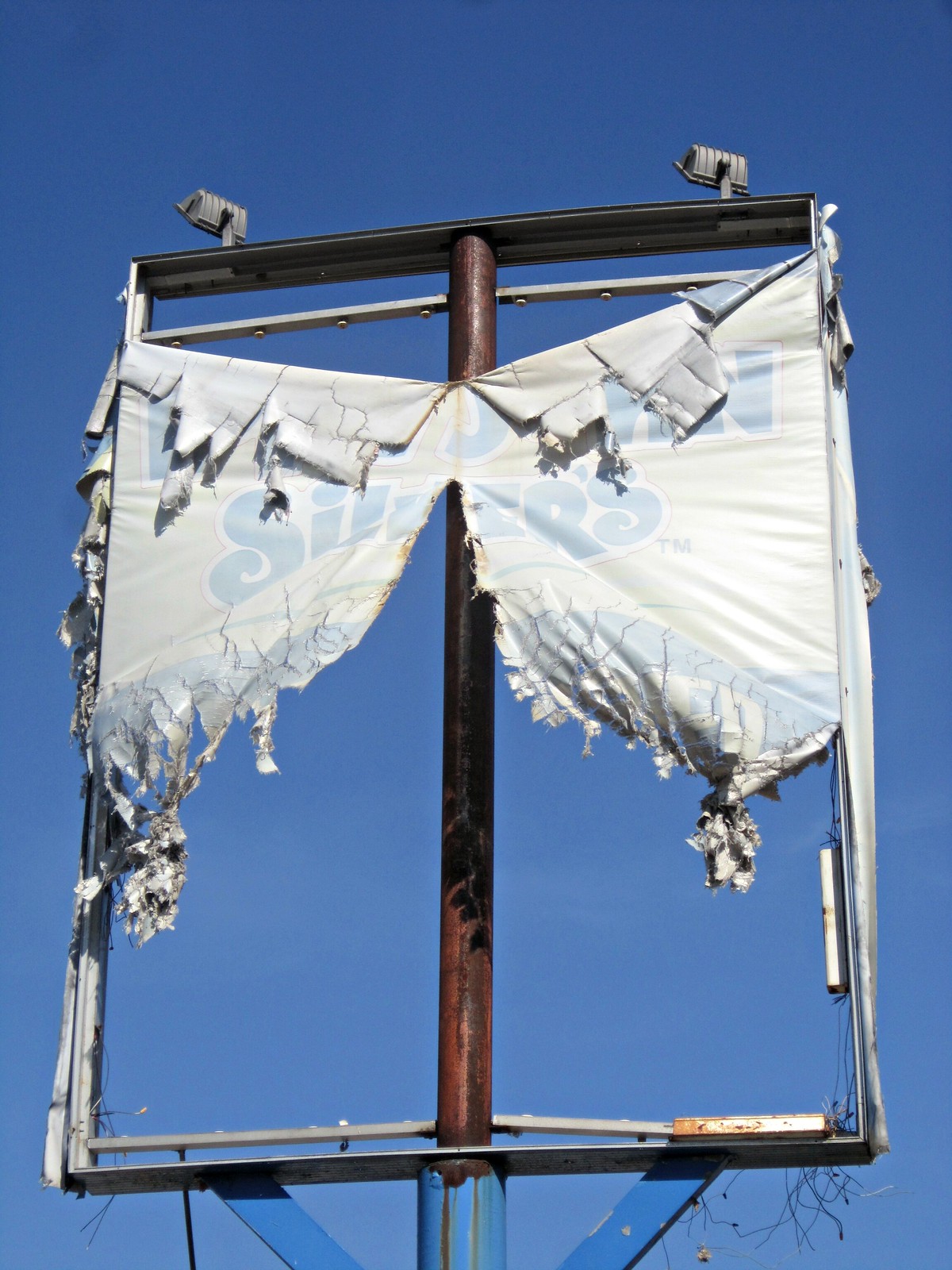A heavily damaged sign for a Long John Silver's restaurant, torn in half and barely legible. The destruction is so extensive that it's difficult to discern the original wording on the sign. An intriguing and unusual sight, capturing the viewer's attention with its dramatic state of disrepair.